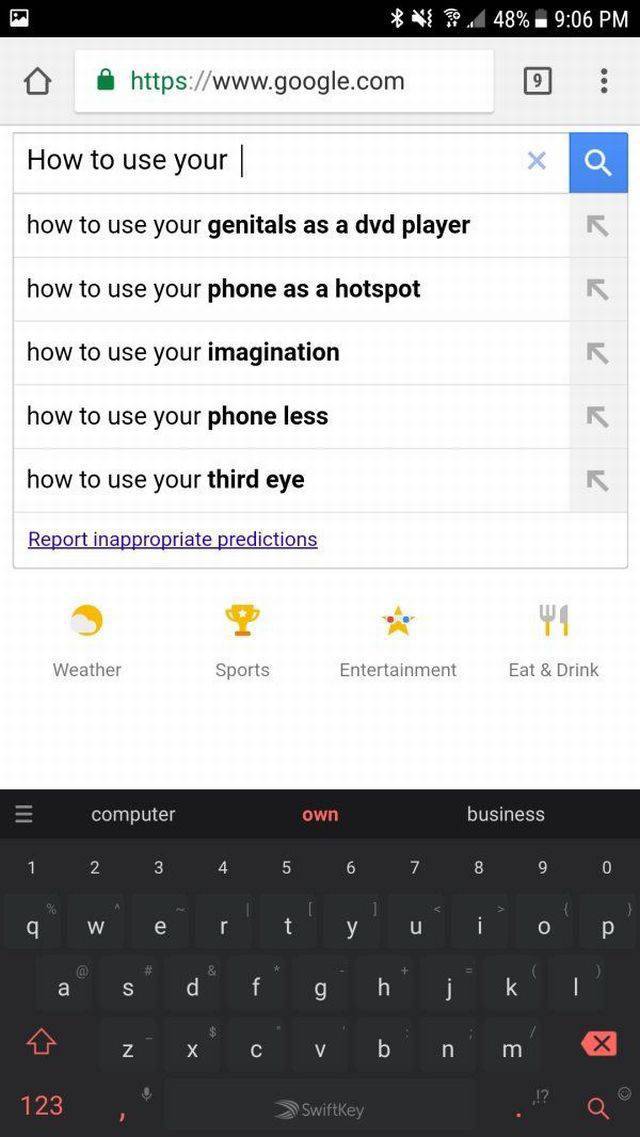The image depicts a Google search page displayed on a mobile phone. At the top of the screen, a black bar features various white icons, indicating the Wi-Fi signal strength, battery level at 48%, and the current time, 9:06 PM. Below this bar, the URL displayed includes "https://" in green, followed by "www.google.com" in gray. Central to the screen is a search bar with a blue microphone icon on the right side. The user's search query reads "how to use your," and the autocomplete suggestions include:

1. How to use your genitals as a DVD player
2. How to use your phone as a hotspot
3. How to use your imagination
4. How to use your phone less
5. How to use your third eye

Beneath these suggestions, the text "Report inappropriate predictions" appears in a lilac-colored, underlined font, indicating a clickable link. Further down the screen, there are icons accompanied by words, likely shortcuts for different categories: a weather icon labeled "Weather," a sports icon labeled "Sports," a star icon for "Entertainment," and a plate and cutlery icon for "Eat and Drink."